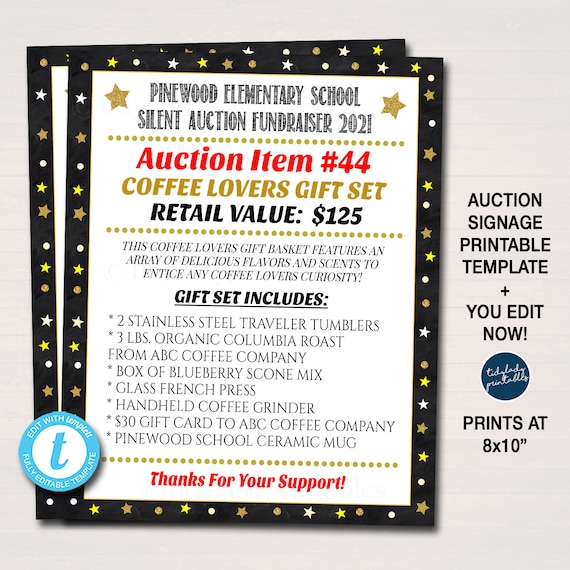This is an 8x10 inch printable auction signage template for the Pinewood Elementary School Silent Auction Fundraiser 2021. The flyer has a white background with a black border adorned with gold and white stars. At the top, between two gold stars, it reads "Pinewood Elementary Silent Auction Fundraiser 2021." Below, "Auction Item Number 44" is prominently displayed in bold red lettering, followed by "Coffee Lovers Gift Set" in gold letters and "Retail Value $125" in black. A section with a gold dotted border provides a detailed description of the coffee lover's set, listing its contents. The flyer concludes with a "Thank you for your support" message. On the left side, there's a blue circle with a T inside, indicating it is a fully editable template.